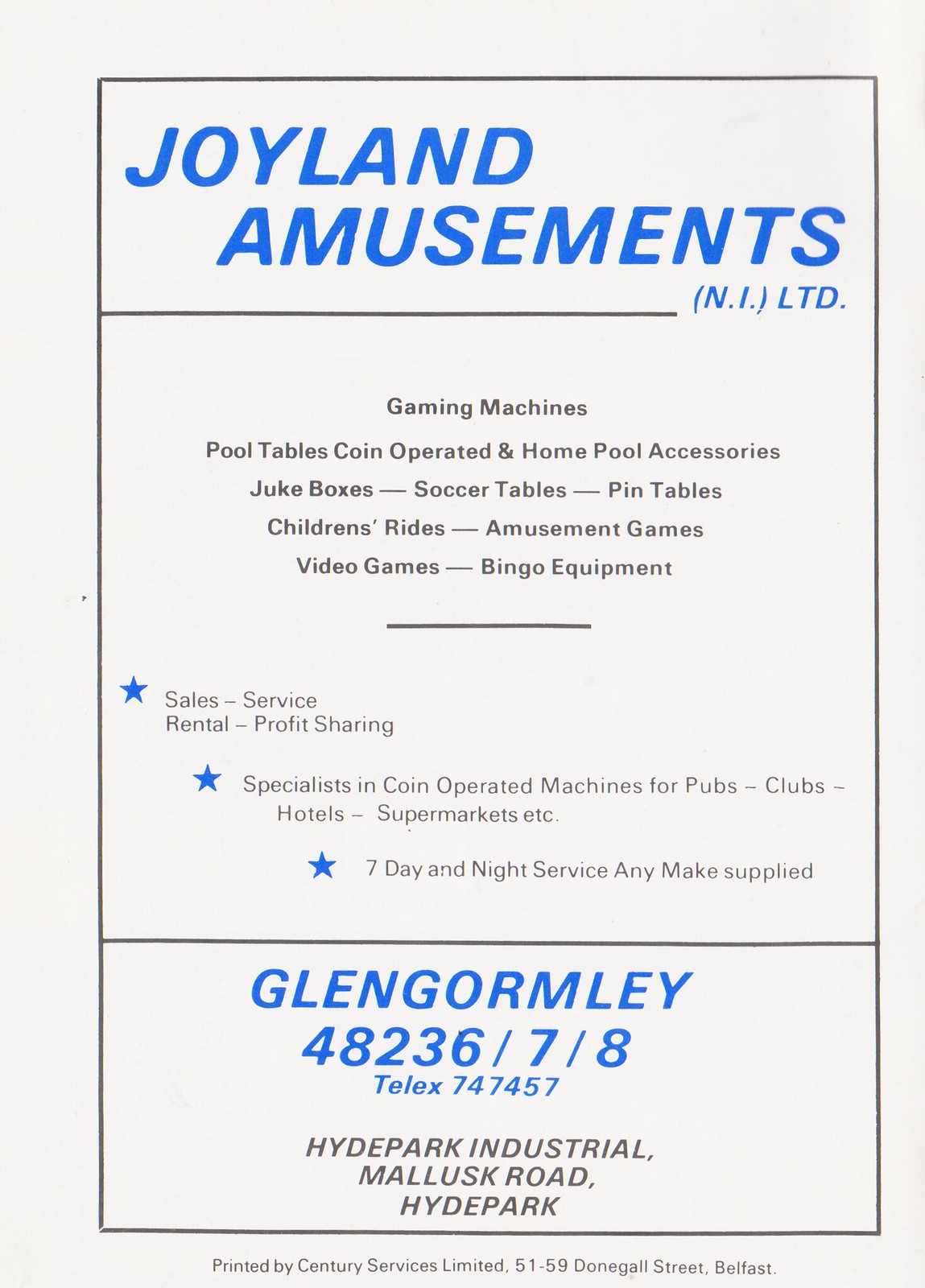The image features a business card or flyer for Joyland Amusements NI Limited. The card has a white background with a black outline and detailed text primarily in blue and black. The top of the card prominently displays "Joyland Amusements NI Limited" in blue letters, followed by a blue line cutting across from the left before it stops towards the right. Below this line, several services are listed in black text, including "Gaming Machines," "Pool Tables," "Coin Operated and Home Pool Accessories," "Juke Boxes," "Soccer Tables," "Ping Tables," "Children's Rides," "Amusement Games," "Video Games," and "Bingo Equipment."

Further down, three blue stars section off additional information:
1. First blue star: "Sales, Service, Rental, Profit Sharing."
2. Second blue star: "Specialists in Coin Operated Machines for Pubs, Clubs, Hotels, Supermarkets, etc."
3. Third blue star: "7-Day and Night Service, Any Make Supplied."

At the bottom in blue text are contact details: "Glen Gormley 4823678," "Telex 747457," followed by the address "Hyde Park Industrial, Malusk Road, Hyde Park." The card notes at the bottom that it was printed by "Century Services Limited, 51-59 Donegal Street, Belfast." Overall, the design uses a blend of blue and black text on a clean white background to deliver an eye-catching and informative advert for the company’s offerings in amusement and gaming equipment.